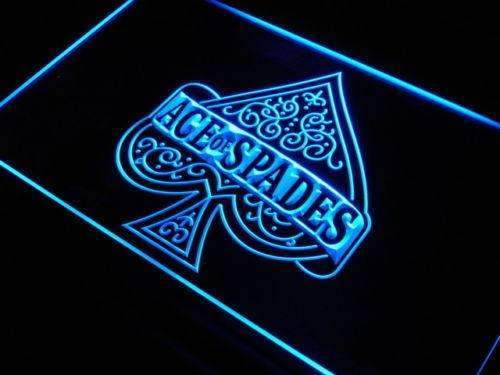This photograph captures what appears to be a neon sign or logo, likely for a nightclub, featuring the iconic spade symbol used in cards. The setting of the image is unknown but the style is distinctly photographic. Dominating the frame is a bright, neon blue spade that inclines diagonally from the bottom left to the top right against a pitch-black background. The spade is intricately detailed with swirling, decorative designs and is enclosed within a rectangular box that is bordered by a thin, bright blue neon line.

Overlaying the center of the spade is a banner in the same neon blue hue that reads "ACE OF SPADES" in bold, black capital letters, evoking a reference to the Motörhead song. This banner curves elegantly around the spade, adding to its ornate appearance. The double-bordered design consists of a blue outline, followed by a black frame, and another inner blue border, which enhances the overall visual impact. The top right corner of the rectangular box appears to be slightly cut off, but this does not detract from the striking effect of the neon artwork against the dark backdrop.